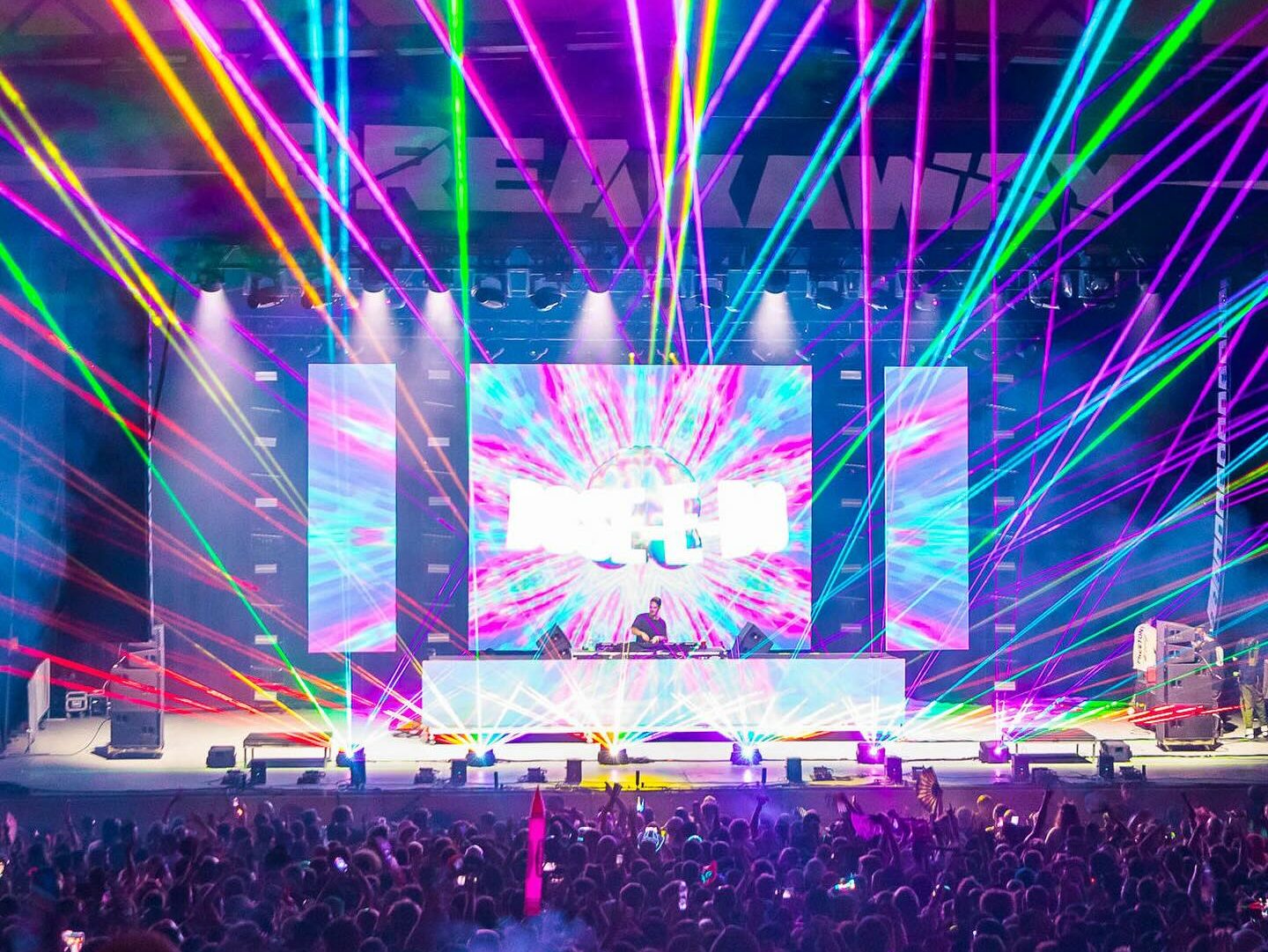The image captures a vibrant nighttime concert scene in a large indoor venue, viewed from a balcony overlooking the stage. The focus is on an artist, standing at a large, rectangular white control panel or desk, which features turntables. The artist is dressed in a black shirt and a hat. The stage is awash with an electrifying display of neon-colored lasers – green, pink, purple, yellow, orange, and blue – that illuminate the dark space. Behind the artist, a central screen displays bright white text, somewhat washed out but with a discernible letter 'E' in the center, framed by additional vertical panels that extend a glowing neon flower pattern in pink and blue. The setting is filled with a massive crowd, backs turned to the camera, many with hands raised or holding luminous objects like smartphones or glow sticks, contributing to the overall iridescent ambiance.